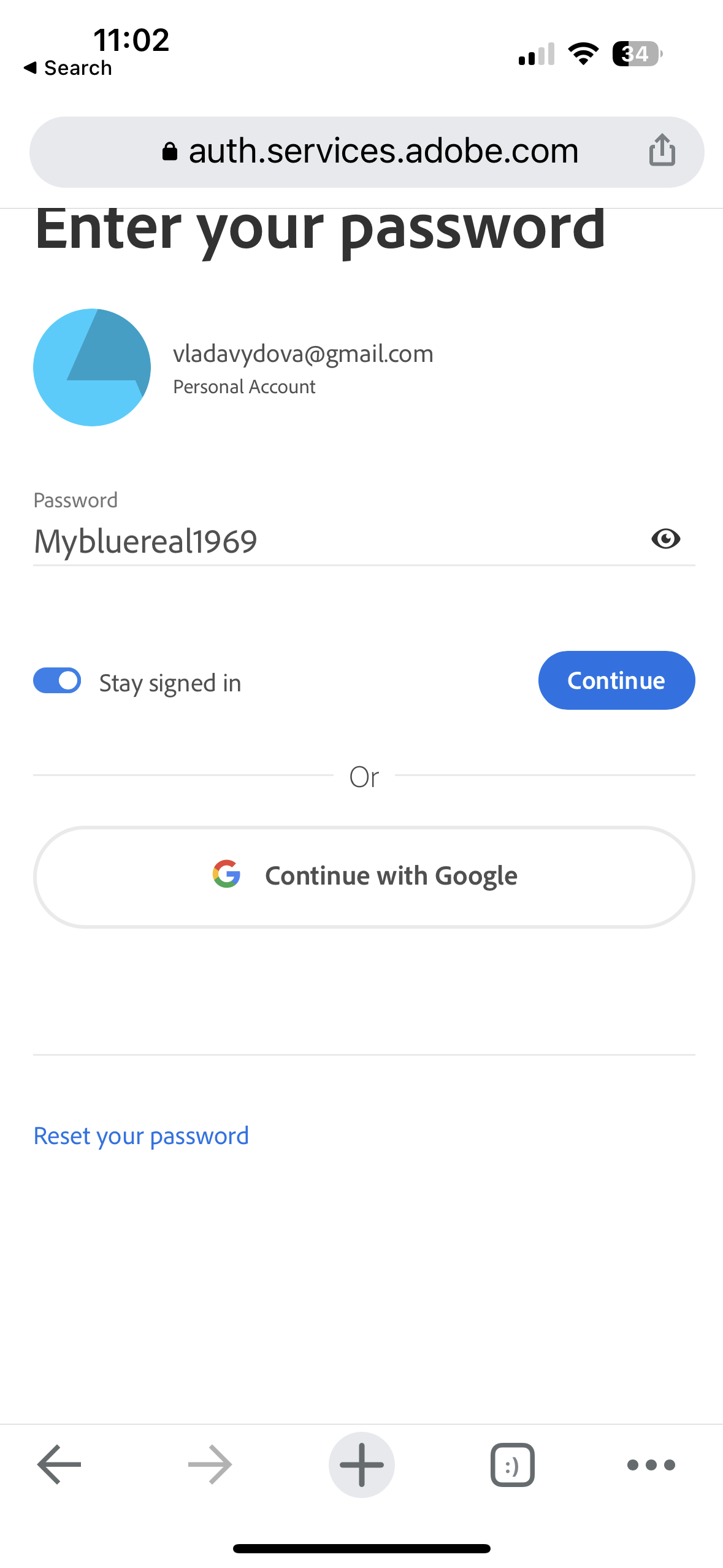The screenshot displays a smartphone authentication screen for an Adobe service. The background is completely white. At the very top, the time is shown as 11:02, accompanied by the status indicators, including two out of four bars for cellular reception, full Wi-Fi signal with three out of three bars, and a battery icon indicating 34% charge. 

Directly below the status indicators, there is a search option, and then a search window with "auth.services.adobe.com" highlighted. 

Below the address bar, there is a prompt in large black letters that reads, "Enter your password." Immediately beneath this, there's a round blue avatar icon beside the email address "vladavdova@gmail.com," labeled as a "Personal account." 

Following this is a password entry field with the password visible, indicated by an eye icon at the end of the field. There is a toggle button to "Stay signed in," which is selected, and adjacent to this is a small blue "Continue" button. 

Further down, there is an option to "Continue with Google." Below this, in small blue letters, is a link to "Reset your password." 

At the very bottom of the screen, there are navigation icons: arrows for forward and back, a plus sign, an emoji icon, and three horizontal dots for additional settings. A thin horizontal black line marks the very bottom edge of the screen.